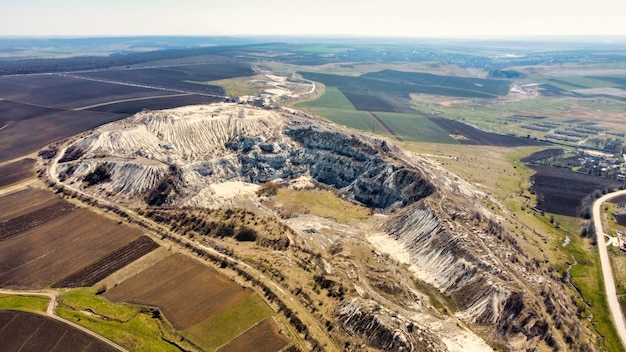The image depicts an aerial view, likely captured from a plane, showcasing an expansive, well-organized farmland with distinct plots. The landscape is predominantly brown with notable patches of green, especially on the right side. The farmlands appear meticulously laid out into rectangular sections, particularly on the left side of the image. In the middle of the photo lies a rugged, mountainous area with flat-topped cliffs and gray rocks, interspersed with some white and brown edges. A large hole is visible in this central mountainous region, suggesting possible excavation activities. The entire scene is topped by a thin, white stripe of sky, emphasizing the vastness of the land below. Multiple roads crisscross the farmland, and on the right side of the image, several buildings cluster together, adding a touch of human activity to the natural and agricultural layout.